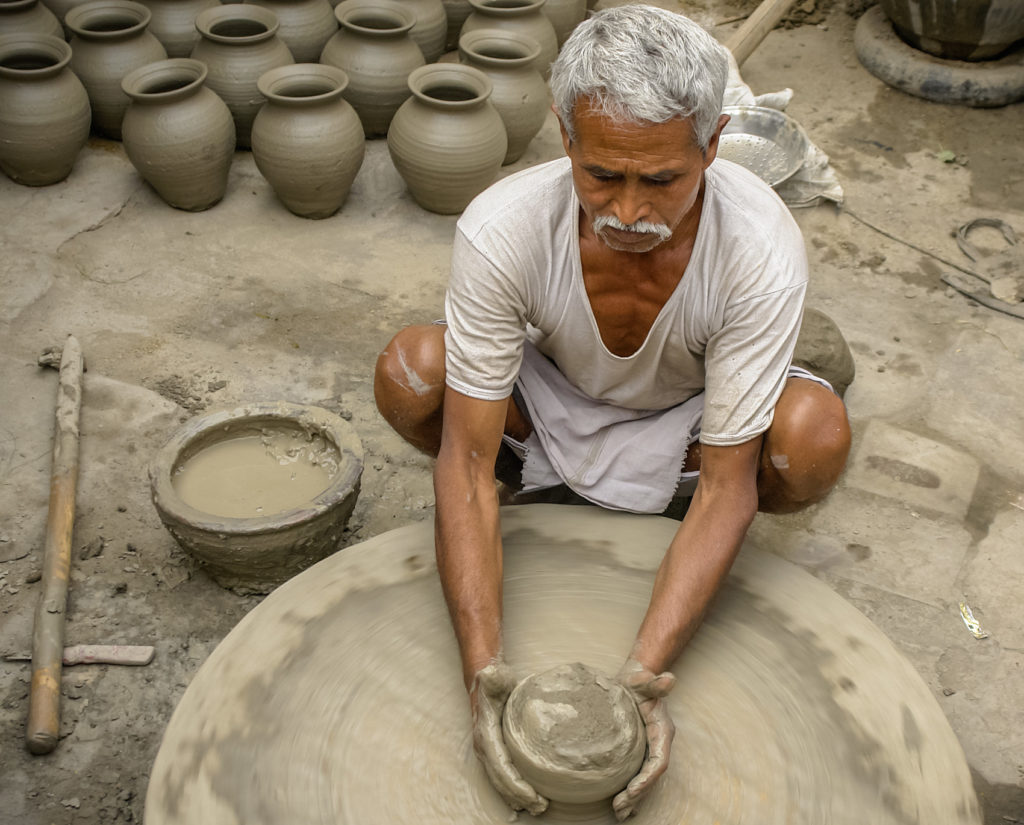The photograph captures an older man with reddish-brown, dark skin, short gray hair, and a gray mustache, crouching down outdoors on a gray cement surface during the daytime. He is wearing a loose-fitting, thin cotton white shirt with a heavily pulled-down collar and white shorts, alongside a white apron. The man is squatted with both knees bent on his heels in front of a large, brown-gray potter's wheel, focused intently as he molds a piece of cylindrical, grayish-beige clay with both hands. His hands are covered in clay as he shapes it on the large spinning stone flat wheel. To his side, there is a clay pot filled with muddy slurry water and a stick covered in clay. In the top left corner of the image, multiple rows of large, thick, gray clay vases, presumably his finished or drying creations, are neatly stacked. The photograph is rectangular, approximately six inches wide and five inches tall, and offers a detailed glimpse into the man's pottery-making process.